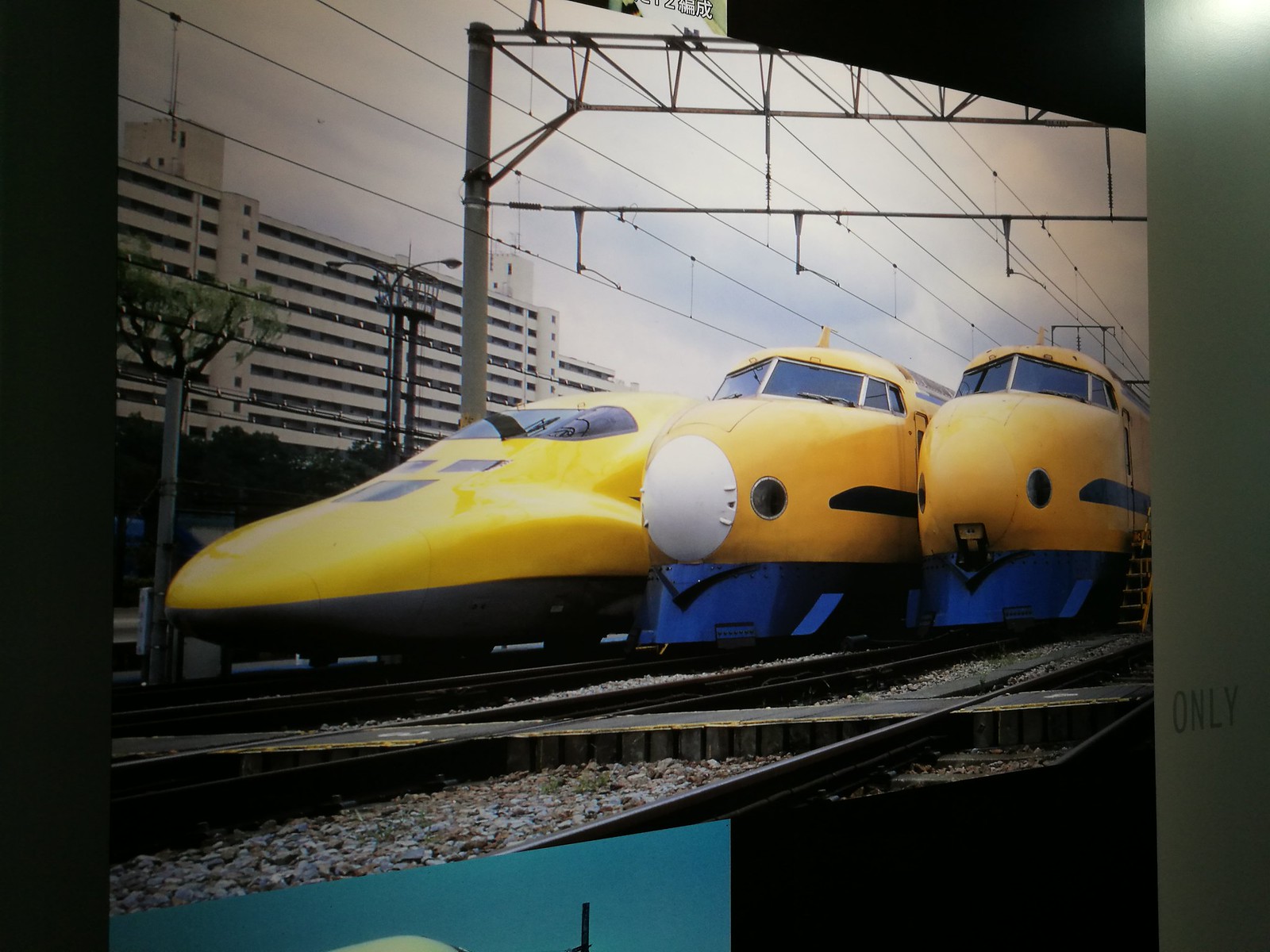The photograph shows an outdoor scene with three high-speed yellow trains positioned side-by-side on the tracks. The train on the far left has a narrow, sleek, and almost bullet-shaped front, indicative of a newer model, with seamless window design. The two trains to the right are older models, featuring more angular window designs. The middle train has a white cap on its nose with small dots alongside, giving it a face-like appearance. All three trains have blue trim along the bottom touching the tracks. The background includes a large white building on the left, several smaller buildings, a couple of trees, and numerous power lines. The ground is covered with gray gravel. Additionally, the photograph appears to be mounted on a white surface with black borders on the left and white borders on the right, casting shadows. The word "only" is written in the bottom right corner of the image.